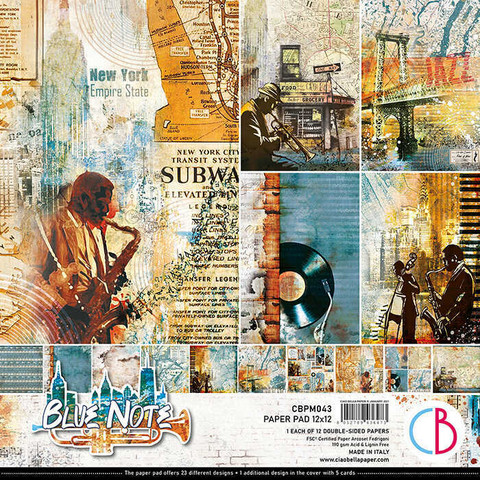The image is an intricate and colorful album cover designed as a collage that merges musical and urban elements. It features multiple squares, each depicting different scenes and objects related to music and New York City. One square showcases a man playing an instrument, possibly a saxophone, while another has an image of a record album. There's a section displaying the iconic Brooklyn Bridge, and another with a man playing a different instrument by a New York-style building. A unique square portrays a record on a player, and another includes a bass and a saxophone player. Prominently, at the bottom, the text "Blue Note" is displayed in white letters against the background of a trumpet and a city landscape. The collage is vibrant, featuring colors such as tan, white, green, blue, light blue, black, purple, pink, and gold, and hints at possible connections to New York culture and music, perhaps serving as either a poster or an album cover. Additionally, a barcode is present on the right, indicating it might be marketed for sale.